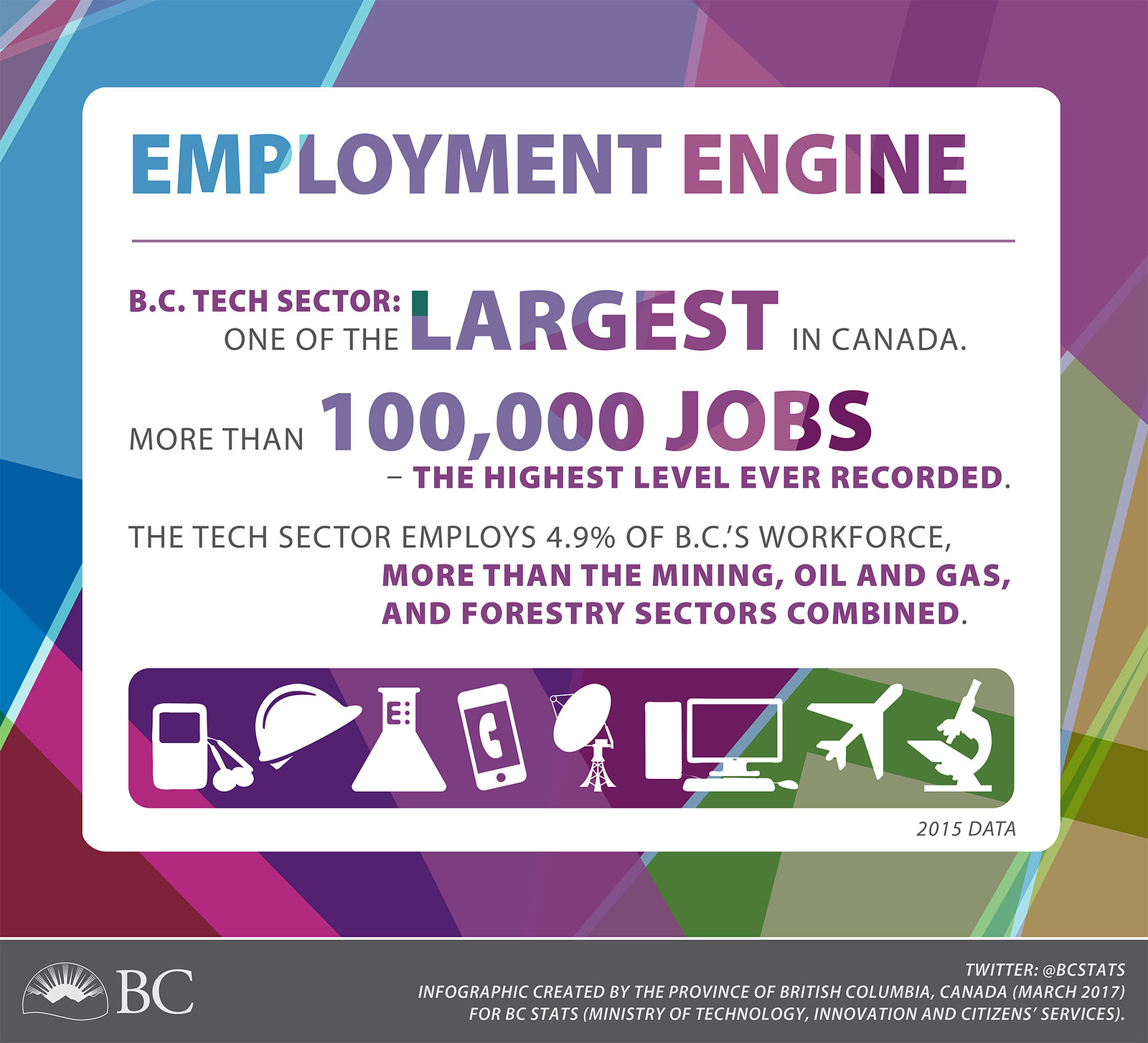The image is an advertisement or informational infographic highlighting the employment landscape of the tech sector in British Columbia, Canada. The background is a vibrant, multicolored design featuring shades of blue, purple, fuchsia pink, and green. At the center of this colorful backdrop is a prominent white box with text that reads: "Employment Engine, BC Tech Sector, one of the largest in Canada, more than 100,000 jobs, the highest level ever recorded. The tech sector employs 4.9% of BC's workforce, more than the mining, oil and gas, and forestry sectors combined." Surrounding the text are various tech-related images, including a hard hat, an airplane, a microscope, a computer, an MP3 player or phone, and a laboratory beaker. At the bottom of the image, a gray box contains the text: "BC Twitter, BCStats. Infographic created by the Province of British Columbia, Canada, March 2017, for BCStats, Ministry of Technology, Innovation, and Citizen Services."